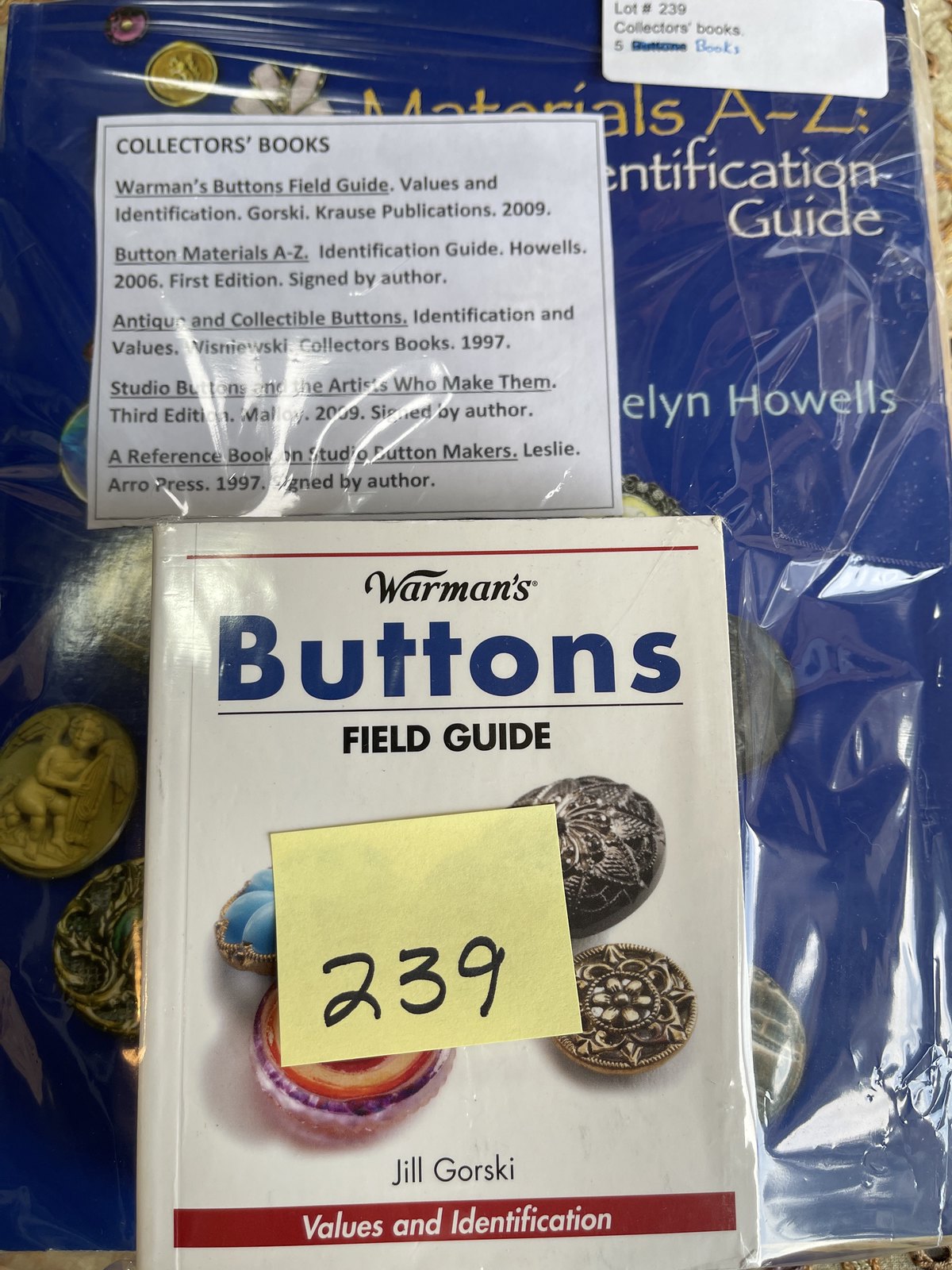The image shows a bundle of collector's books meticulously wrapped in plastic. At the top left of the package, there is a white slip of paper with printed black text, though the reflection of the light on the plastic makes it difficult to read clearly. The paper lists several works: "Collector's Book: Warman's Buttons Field Guide, Values and Identification, by Gorky, Krauss Publications, 2009"; "Button Materials A-Z Identification Guide by Howells, 2006, First Edition, Signed by the Author"; and "Antique and Collectible Buttons: Identification and Values by Viennese, Key Collector's Book, 1997." Additionally, a yellow sticky note with "239" indicates the lot number, hinting this is a compiled prize package. Prominently visible on top is "Warman's Buttons Field Guide" with the author's name, Jill Gorski, mentioned below, emphasizing values and identification.